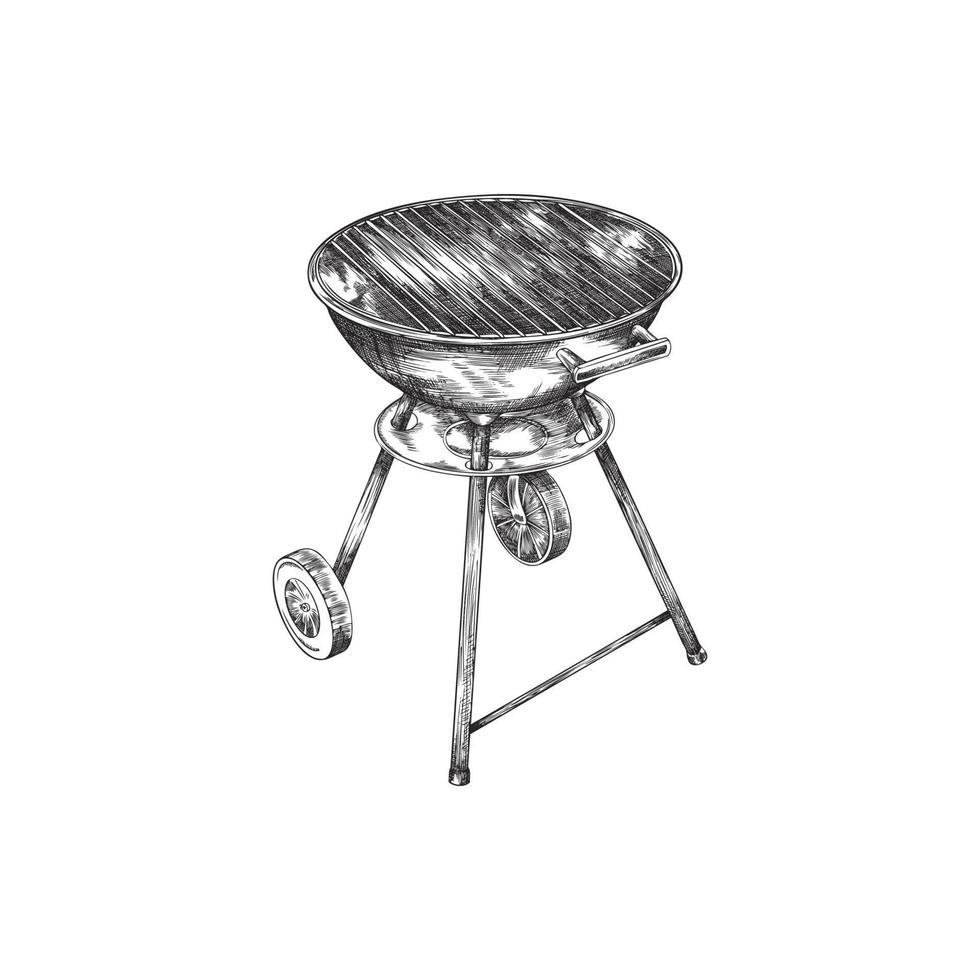The image is a highly detailed pencil or charcoal drawing of a small, round charcoal grill. The grill has a circular bowl on top, covered with a metal grate. Below this bowl, there is a smaller catching tray meant to catch spills or oil. The grill’s structure is supported by four legs: the front two legs have small wheels, allowing the grill to be easily moved, while the back two legs are stationary metal poles connected by a crossbar for added stability. The bowl's surface is depicted as shiny, with noticeable reflections both inside and on the lip. The handle attached near the top allows for the grill to be pulled or pushed conveniently. The wheels include meticulously drawn spokes, enhancing the overall detailed and realistic appearance of the sketch. The scene lacks any background, giving the impression of a freehand drawing focused solely on the grill itself.